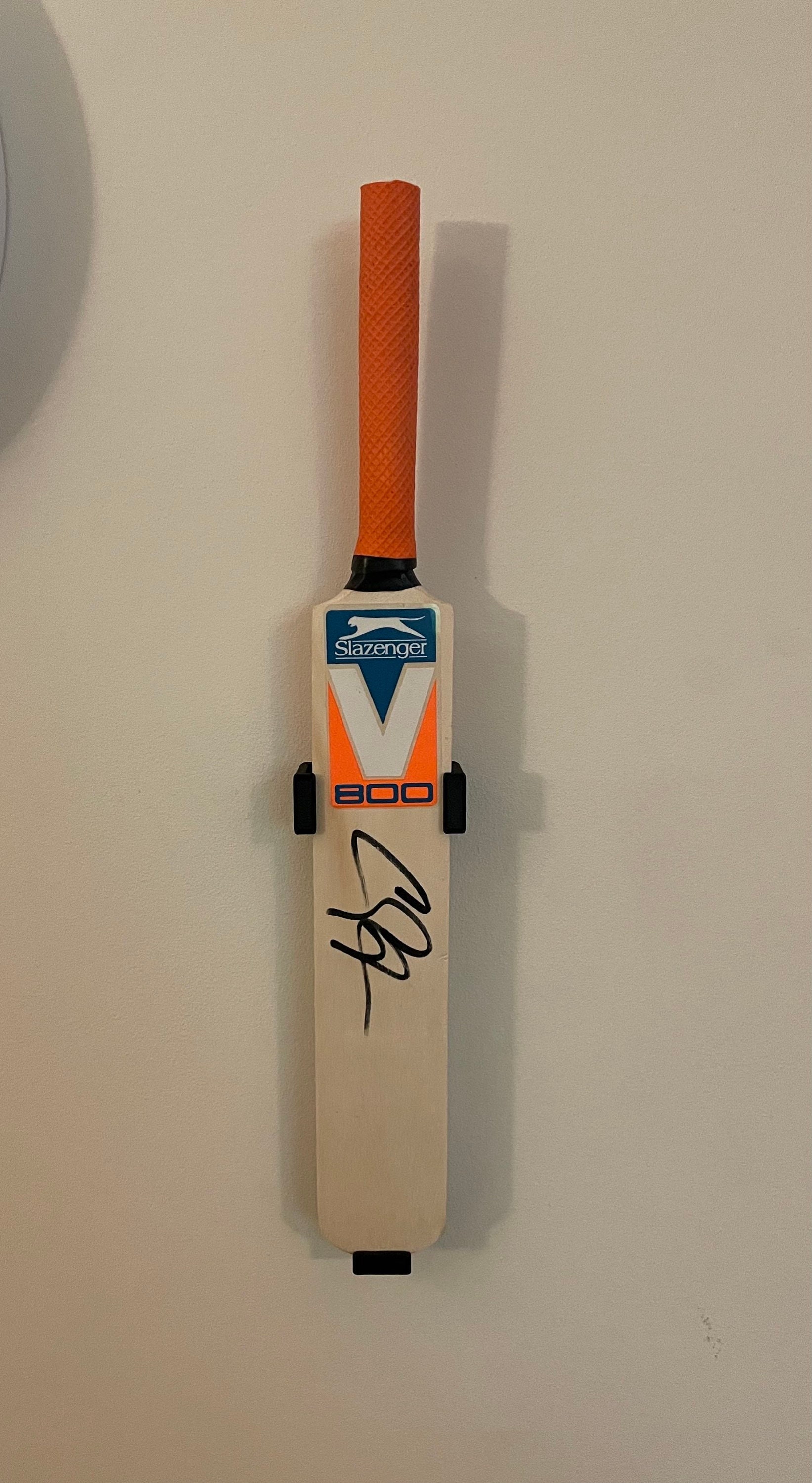This is a photograph of a tan wooden cricket bat mounted vertically on a white wall using black brackets. The bat features an eye-catching bright orange handle with a crosshatched grip for better hold. The handle is connected to the bat with a black band. Below the handle, a blue rectangular label is affixed, adorned with the logo of a running puma or cougar and the name "Schlesinger." The label includes a prominent white "V" with silver outlining, and underneath it in black letters on an orange background, the number "800." The bat has been autographed with illegible initials in black permanent marker, adding a personal touch to it. A slight shadow of the bat is cast onto the wall, giving the image a subtly dynamic dimension.